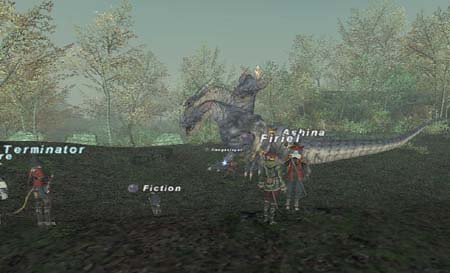In this detailed screen capture from a multiplayer RPG, the scene presents a dark bluish-gray sky, suggesting either an overcast day or a late afternoon in the game world. The backdrop features a row of green-leaved trees, with the closest tree displaying some brown highlights. The uneven ground beneath the characters is a mixture of dark stone and dirt, creating a dramatic setting for the unfolding action. In the foreground, a group of characters, dressed in medieval or Renaissance clothing, stand on a dark green hill that slopes from left to right. Their names—Terminator, Fiction, Fire, Ashina—are displayed in white above their heads. Behind these characters, a menacing dark gray dragon looms, seemingly preparing to attack. The scene is framed by additional hills on the right side, where more trees grow, reinforcing the sense of an expansive and mysterious game world.